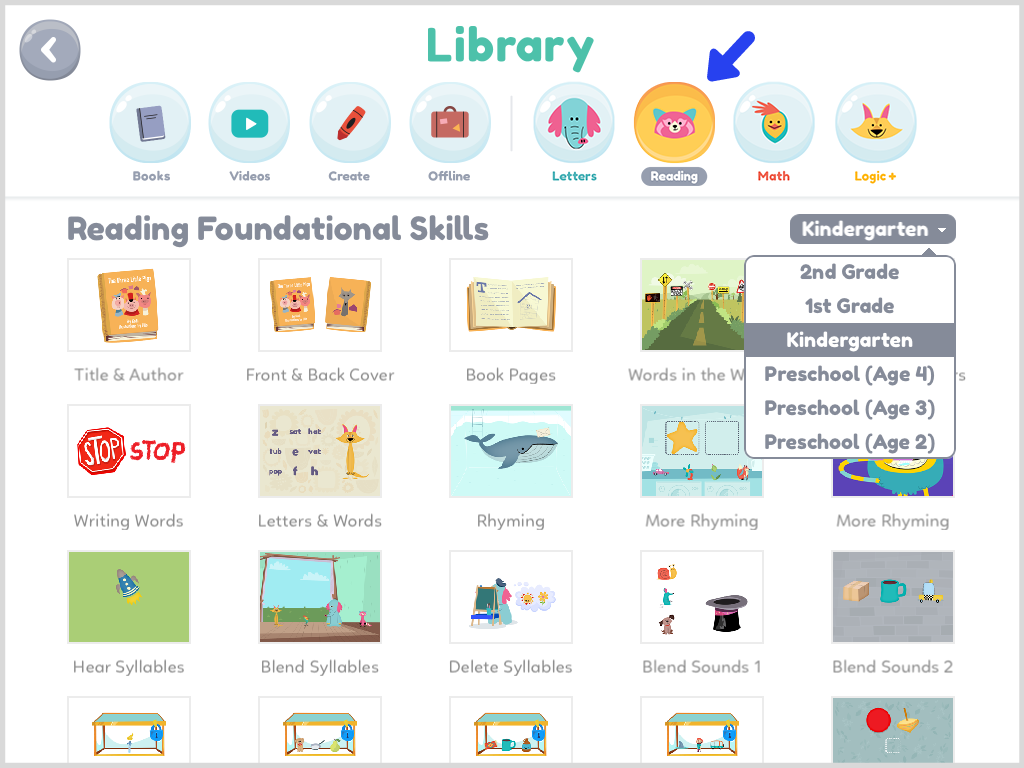The image is a detailed layout of an educational library interface. At the top center, the word "Library" is prominently displayed in a greenish hue. In the top left corner, there is a white arrow pointing left, encased in a circular gray background. The top middle section features four bubbles on both the left and right sides. The left bubbles are labeled "Books," "Videos," "Create," and "Offline," while the right bubbles are tagged "Letters," "Reading," "Math," and "Logic."

Below this section, on the left side, the heading "Reading Foundation Skills" is visible. This segment contains multiple squared boxes with images and corresponding labels. The first row displays four boxes, labeled "Titles and Author," "Front and Back Cover," "Book Pages," and "Words and the W." The second row consists of five boxes, labeled "Writing Words," "Letter and Words," "Rhyming," and two boxes labeled "More Rhyming." The third row showcases another set of five boxes, labeled "Syllables," "Blend Syllables," "Delete Syllables," "Blend Sounds One," and "Blend Sounds Two."